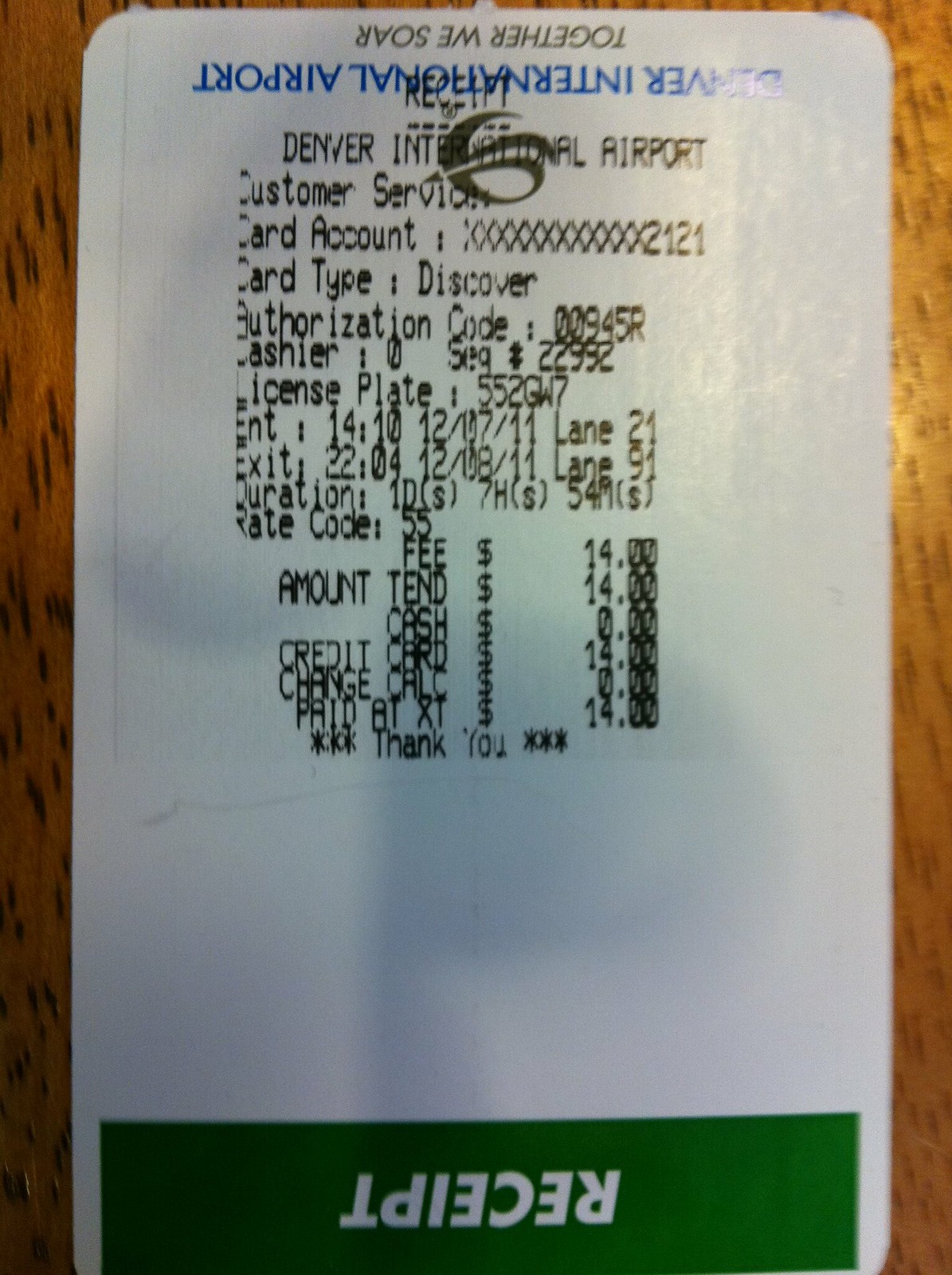This image is a close-up shot of a receipt from the Denver International Airport. The receipt itself is printed on white paper. At the bottom of the ticket, a green bar with white letters displaying the word "RECEIPT" appears upside down. Above this green bar, "Denver International Airport" is printed.

At the top of the receipt, it reads "Together We Saw" in black letters with blue ink.

The detailed printout on the receipt includes the following information:

- "RECEIPT: Denver International Airport Customer Service"
- "Card Account **** 2121"
- "Card Type: Discover"
- "Authorization Code: 00945R"
- "Cashier: 0"
- "Sequence: 22992"
- "License Plate: 552GW7"
- "Entered at: 14:10 on 02/07/2011"
- "Lane: 21"
- "Exited at: 22:04 on 02/08/2011"
- "Lane: 91"
- "Duration: 1 day 7 hours 54 minutes"
- "Rate Code: 55"
- "Fee: $14"
- "Amount Tendered: $14"
- "Cash: $0"
- "Credit Card: $14"
- "Change Calculations: $0"
- "Paid at XT: $14"

At the bottom of the receipt, it says "Thank You," flanked by three asterisks on each side (*** Thank You ***).